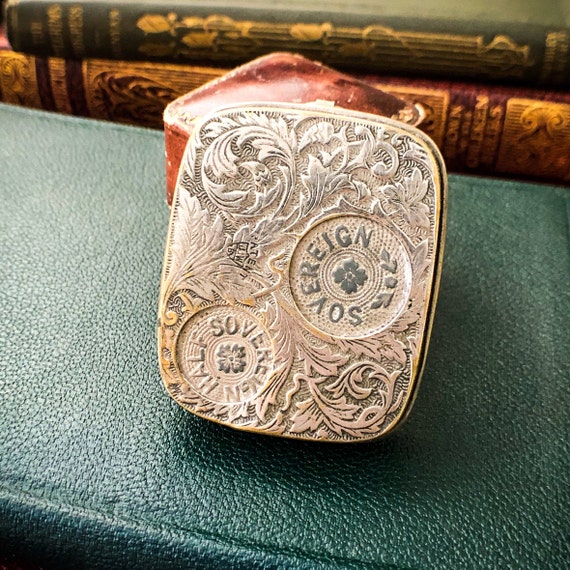This professionally taken close-up photo features an intriguing metallic object with ornate, scrolling organic leaf and vine engravings, leaned against a worn brown leather box. The object, possibly a compact mirror or lid of a metal box, appears old and well-used, displaying a silver finish with areas of green patina in worn crevices. Central to its design are two circular engravings, one reading “Half Sovereign” and the other “Sovereign,” hinting at its historical or monetary significance. The object is positioned on the spine of an elegant green leather-bound book, set against a backdrop of additional vintage books—one green and one red, both adorned with gold embossing. This detailed arrangement contributes to the photograph's rich, antiquarian ambiance.